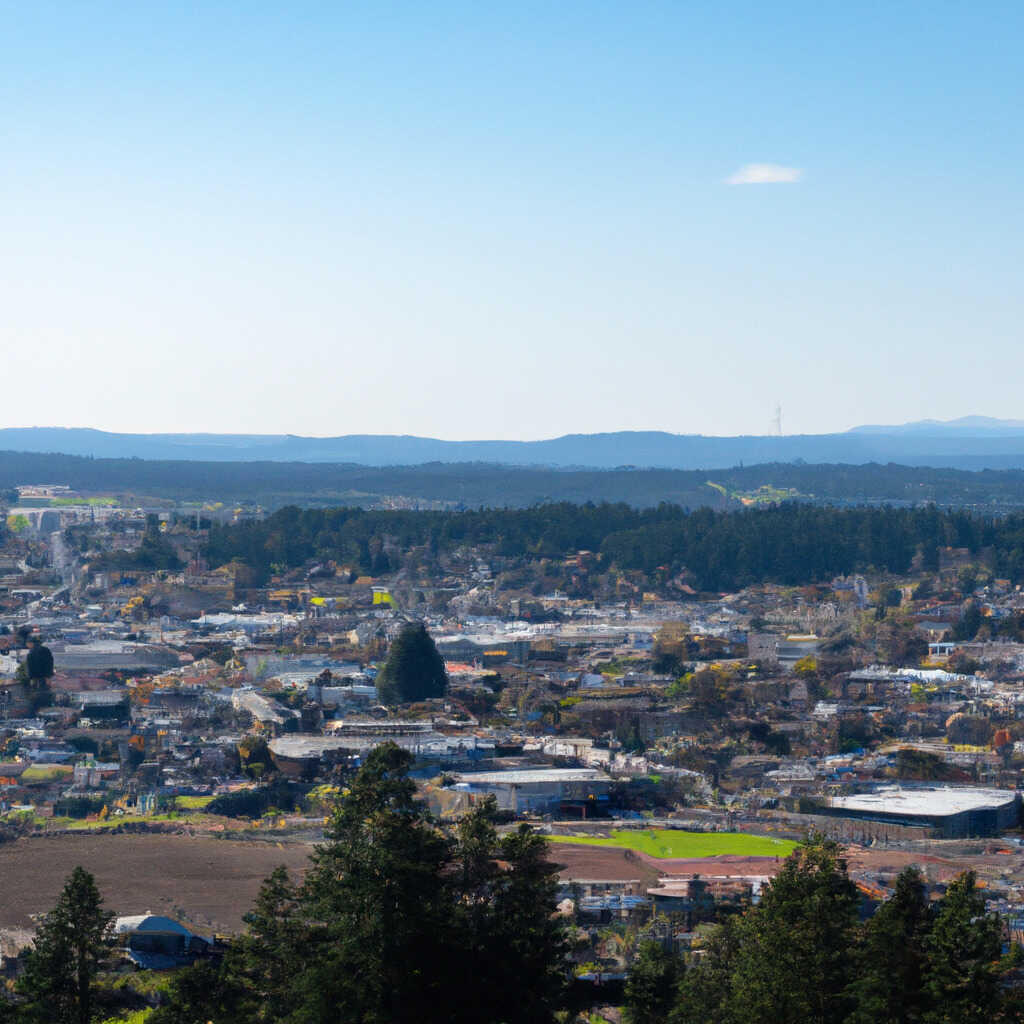The image depicts a seemingly serene small city, possibly situated on either the East or West Coast of the United States. In the distant background, a range of majestic mountains creates a captivating contrast against the bright blue sky, which is mostly clear except for a lone, fluffy white cloud. The city's lush greenery suggests a summer season, with various types of trees that may either be evergreen or deciduous, yet it’s difficult to determine based on this image alone.

In the foreground, there's evidence of a recreational area, which could plausibly be a golf course or a baseball field. Despite the natural beauty and tranquil setting, the city itself appears to be in a state of disrepair. The infrastructure looks neglected, with buildings and other structures seemingly deteriorating, evoking an overall impression of abandonment or prolonged neglect rather than the aftermath of a natural disaster.